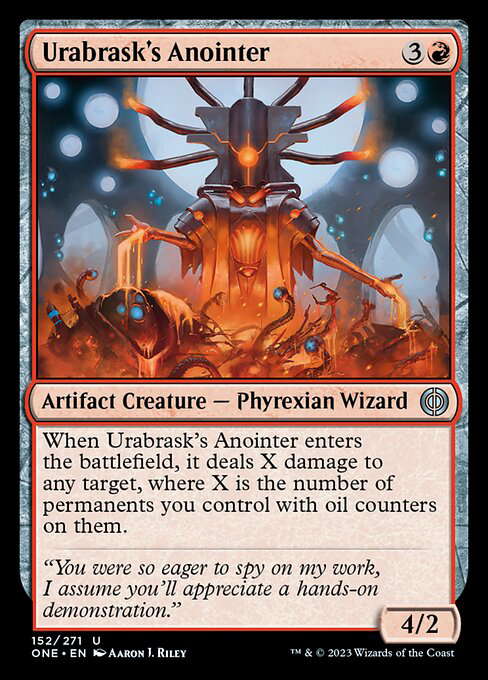This image is a detailed close-up of a Magic: The Gathering playing card titled "Eurabrask's Anointer." At the top of the card, set within a beige background with a red outline, are the words "EURABRASK'S ANOINTER" in black text and a circle containing the number three and a black fireball icon. The depicted creature appears to be a metallic, insectoid being, primarily gray with orange accents. It has two arm-like appendages and a steel-like headpiece featuring seven appendages, each tipped in orange. The creature is surrounded by other entities that seem to be engulfed in flames. Below the illustration, the card reads in black text: "Artifact Creature — Phyrexian Wizard." The card's ability is detailed as follows: "When Eurabrask's Anointer enters the battlefield, it deals X damage to any target, where X is the number of permanents you control with oil counters on them." Additionally, there's a flavor text quote: "You were so eager to spy on my work. I assume you'll appreciate a hands-on demonstration." At the bottom of the card, the details include the numbers "152/271" on the left and "4/2" on the right, along with the illustrator's name, Aaron L. Riley. The card also features a trademark and copyright note: "© 2023 Wizards of the Coast."